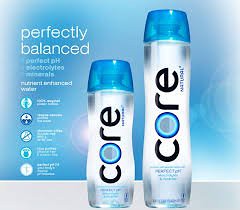This is a low-quality screenshot of an advertisement for Core Natural Water. The image features two bottles with the brand name "Core" written vertically in black letters, with the 'O' depicted as a multi-shaded blue circle. The bottles have white bases and blue caps. The taller bottle is on the right and is a standard size, while the smaller bottle, which is about 75% the size of the larger one, is on the left and has a more contoured, curvaceous shape. The ad includes text that reads "Perfectly Balanced, Perfect pH, Electrolytes, and Minerals," along with five icons next to these descriptions, although they are too blurry to decipher clearly. One identifiable icon is a test tube with a prohibition sign over it. The ad also employs a color scheme primarily consisting of blue, white, and black.